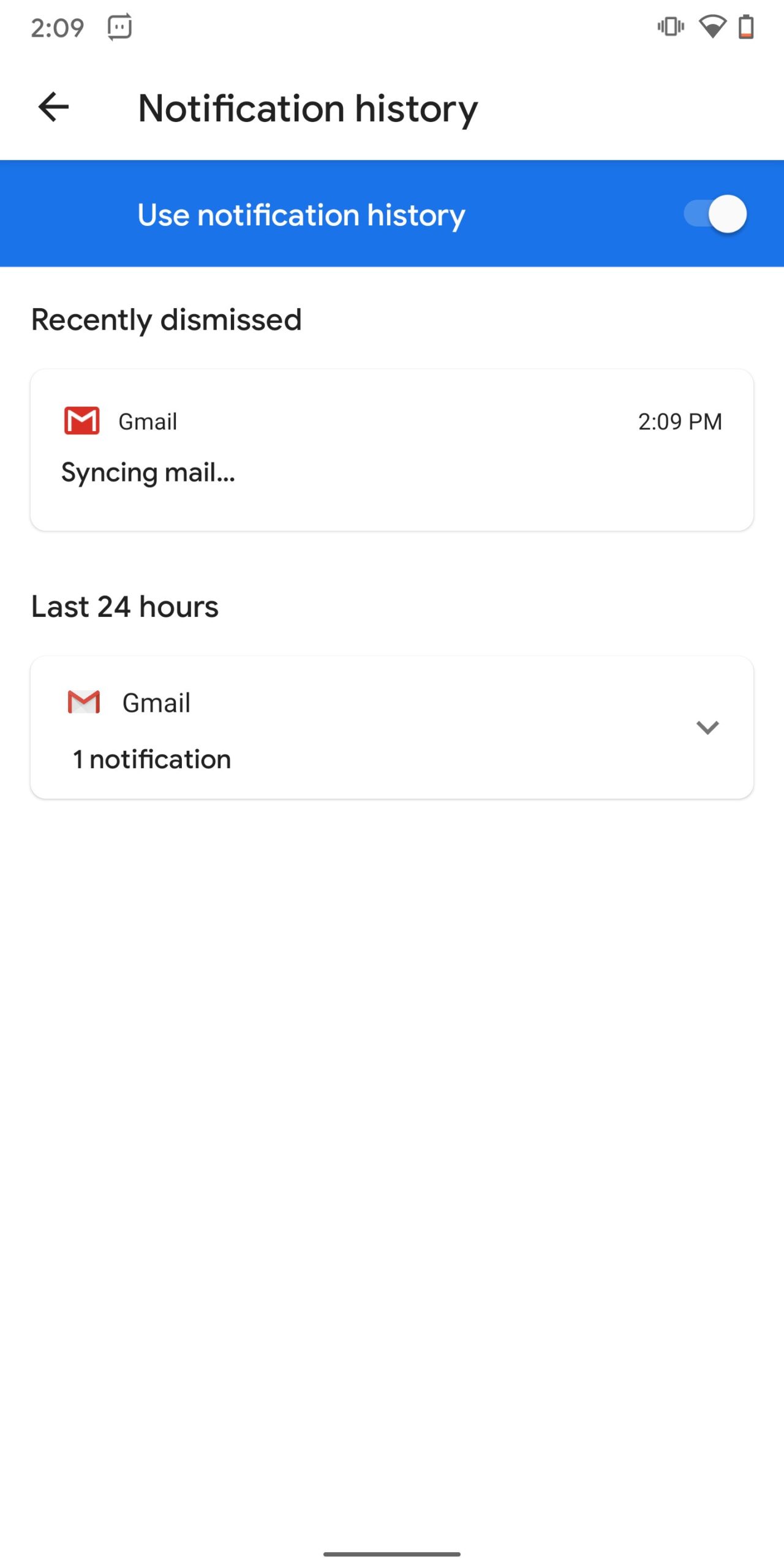The rectangular, vertically-oriented image appears to be a screenshot taken from a cell phone's display. At the very top of the screenshot, a white background shows the time as "2:09 PM" alongside various status icons. From left to right, these icons include a text message icon, a vibrate mode symbol, Wi-Fi connectivity status, and a battery indicator that shows a critically low battery level.

Below this status bar, on the left side of the screen, there's a back arrow icon. To the right of the back arrow, the label "Notification History" is prominently displayed.

Directly beneath "Notification History," a blue banner featuring white text is visible. The banner reads "Use notification history," and adjacent to this text is an active toggle switch indicating that the feature is currently enabled.

The majority of the remaining screen area transitions back to a white background. Here, a section labeled "Recently dismissed" can be seen, which lists "Gmail: Syncing mail" under it, marked with the same time stamp of "2:09 PM." Further down, under the section titled "Last 24 hours," it shows "Gmail: 1 notification," annotated with a dropdown arrow on the right side, suggesting additional details can be expanded.

Overall, the screenshot captures a detailed view of the notification history settings on a cell phone, with particular emphasis on recent Gmail notifications.